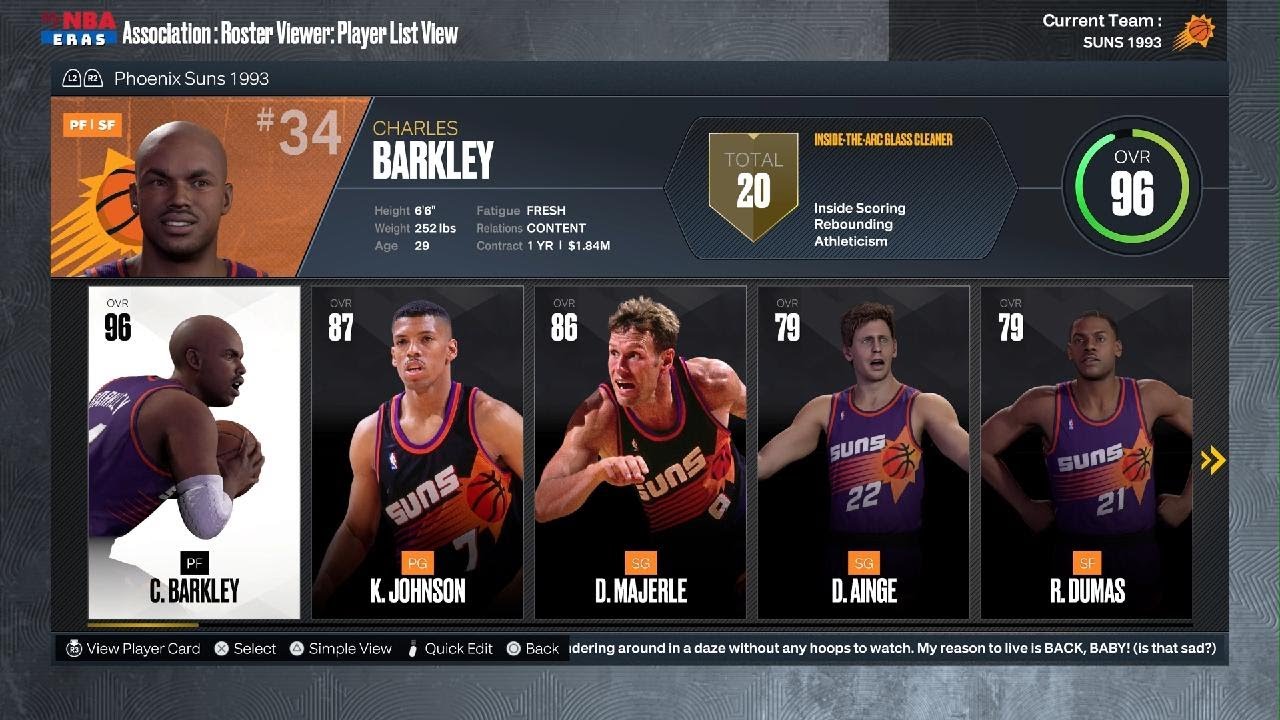This image is a detailed screenshot from a website featuring a virtual basketball game interface, likely related to an NBA-themed game. At the top of the screen, the header "NBA" is prominently displayed in red text. Below this, a blue and white banner features the word "ERAS" in all capital letters. Further down, white text reads: "Association: Roster Viewer: Player List View".

On the right side of the interface, the current team is identified as "Suns 1993" next to a basketball graphic. Beneath this, in white print, it states "Phoenix Suns 1993". There is an orange background with a basketball design behind a prominent number "34", accompanied by a graphic of a player.

To the right of this, the player's name, "Charles Barkley", is displayed, along with detailed information about his height, weight, age, fatigue, relationships, and contract. Additionally, it lists attributes like inside scoring, rebounding, athleticism, and a key rating labeled "OVR 96" enclosed in a green circle.

At the bottom of the screen, a graphic showcases five different players, possibly indicating team members or related stats.